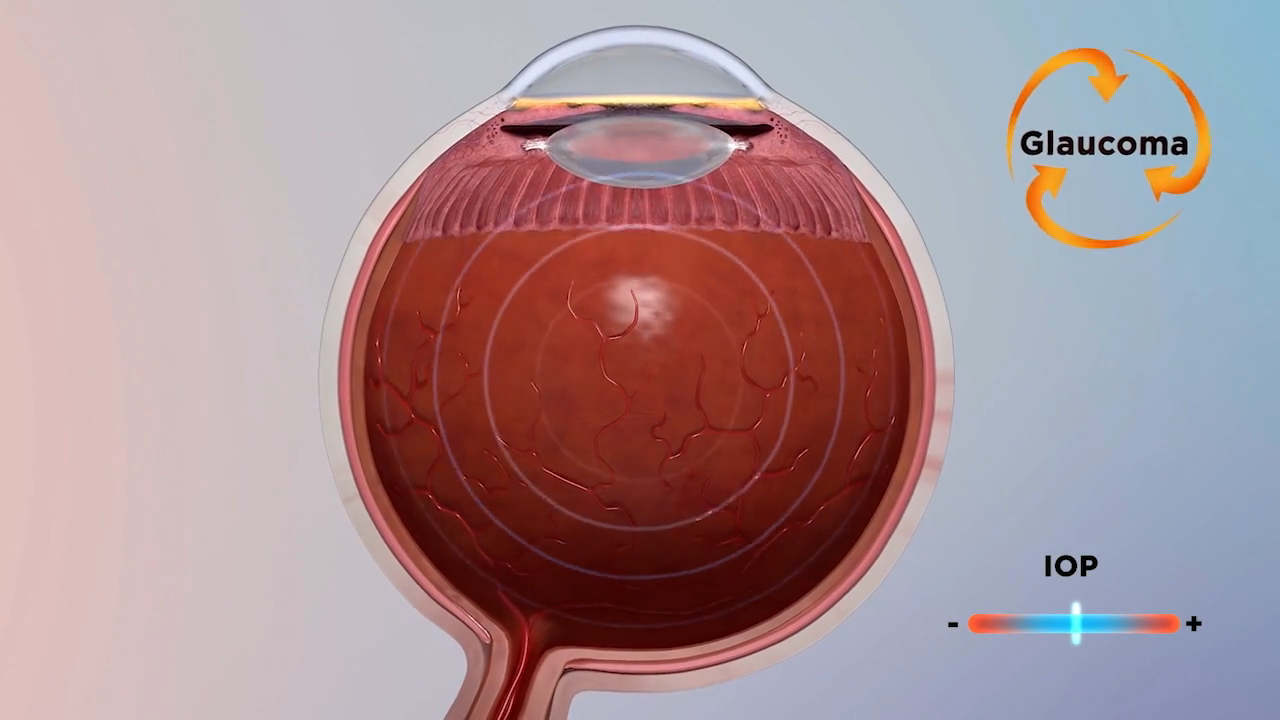This detailed digital anatomical image provides a side view of the human eye, focusing on an eyeball prominently colored red, indicating the presence of blood vessels. Central to the image is the eyeball, showcasing structures such as the lens and cornea located near the top and the optic nerve extending from the bottom. The eye appears filled with a red liquid, symbolizing blood flow. In the upper right corner, a cycle symbol with arrows forms a circle around the word "glaucoma," illustrating the condition's impact on eye health. The lower right corner features a scale marked "IOP" (Intraocular Pressure), with positive and negative indicators flanking a bar, hinting at the variations in pressure measurement. The image, with its circular design and vibrant colors, aims to educate on glaucoma and its effects on the eye.